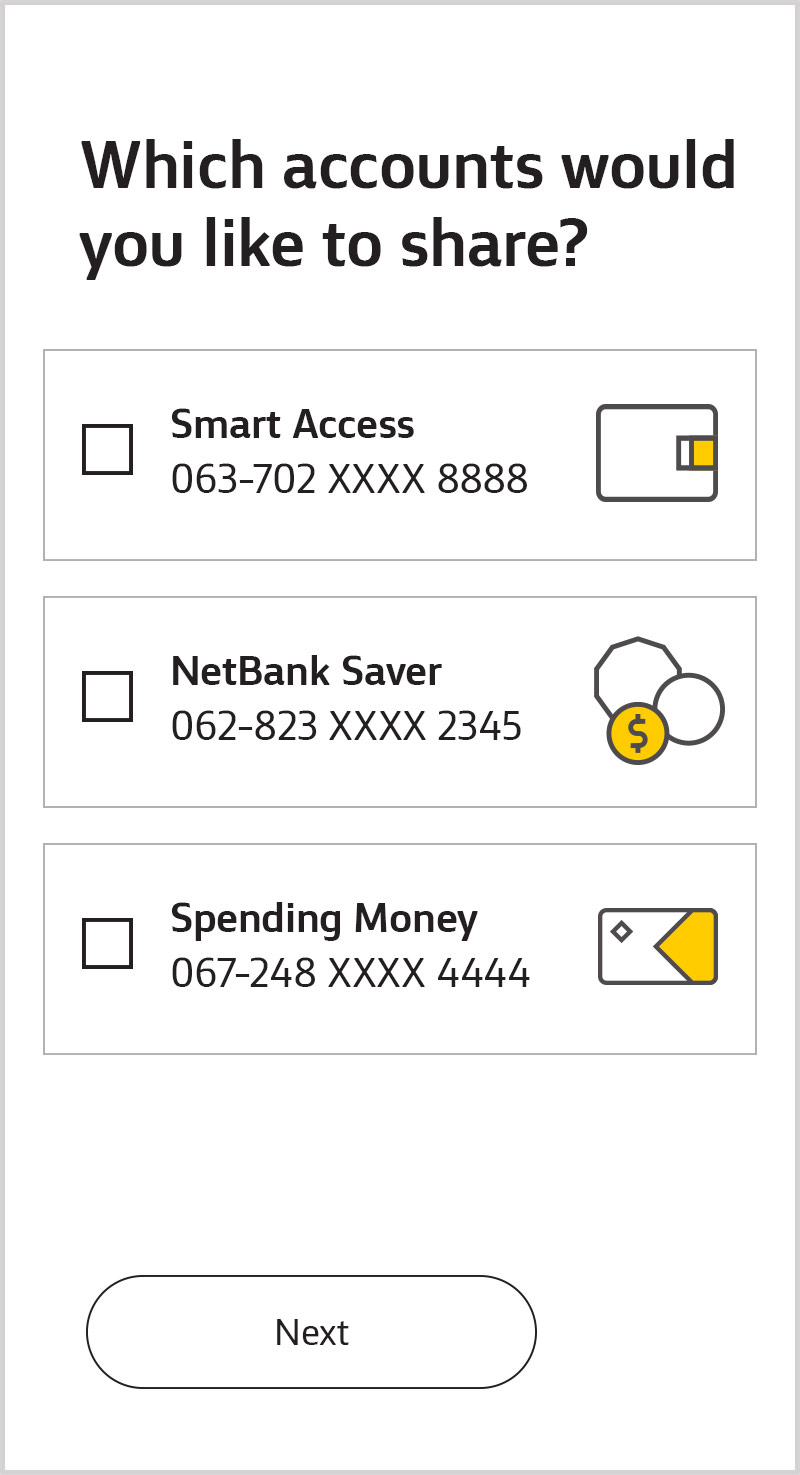The image is an enlarged screenshot from a cell phone interface. The main focus is a vertically oriented white box, prominently placed within a gray frame, resembling the proportions of a smartphone screen. At the top of the box, there is a large text header spread across two lines in bold black letters that reads: "Which account would you like to share?" 

Below this header, there are three horizontal boxes, stacked one above the other. Each box is wider than it is tall and includes a selectable square checkbox on the left side. The first box, labeled "Smart Access," displays a long, unidentified number sequence next to an icon resembling a credit card. The second box, labeled "NetSaver," also includes a long numerical sequence and features an icon depicting three circular shapes, one of which is an octagon-like figure. This icon contains a blank circle and a smaller yellow circle with a dollar sign in it. The third and final box is labeled "Spending Money," accompanied by another unrecognized long number and an icon similar to a credit card.

None of the checkboxes in the three horizontal boxes are currently selected.